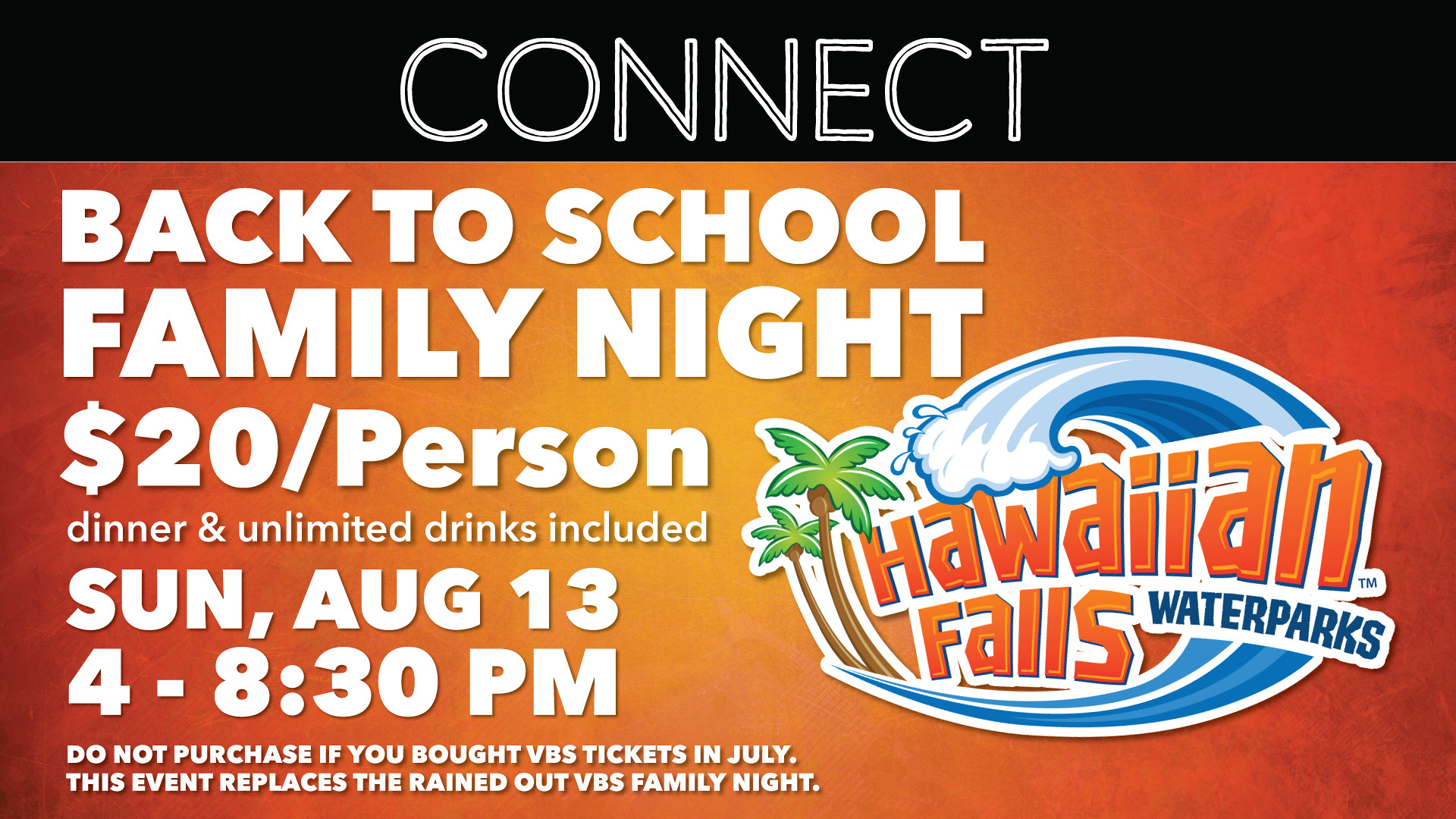The advertisement for Hawaiian Falls Water Parks prominently features a vibrant, eye-catching design geared towards promoting its Back-to-School Family Night event. The top of the image displays the word "Connect" in bold, white letters against a sleek black background. Below this, the main body of the ad showcases an orange backdrop with the event details in bold white text. It announces "Back-to-School Family Night" with a cost of $20 per person, which includes dinner and unlimited drinks. The event is scheduled for Sunday, August 13th, from 4:00 to 8:30 p.m. A special note advises not to purchase tickets if one had already bought VBS tickets in July, as this event replaces the rained-out VBS family night. The image is colorful, clear, and inviting, effectively conveying all necessary information for attendees.